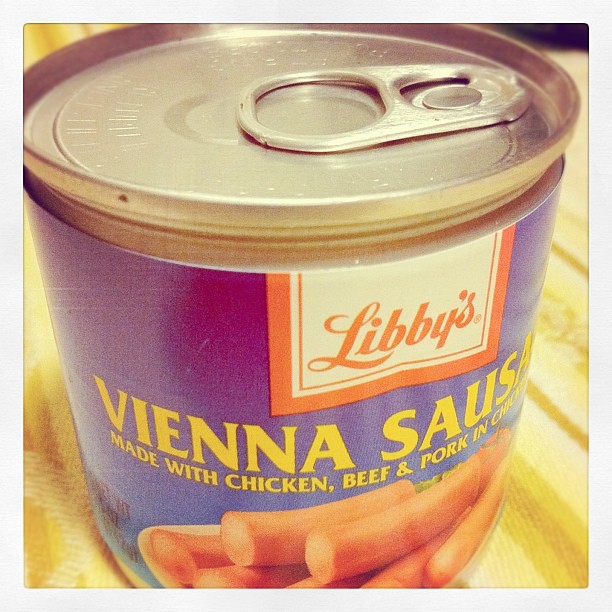The image features a close-up view of a slightly taller-than-wide can of food, viewed from a slightly elevated angle, giving it a foreshortened appearance. At the top of the can, the lid is visible with a metal pull tab positioned on the right-hand side. The branding on the can reads "Libby's" in a distinctive white and red logo. Below the logo, the text "Vienna Sausage" is prominently displayed, indicating the contents as sausages made with chicken, beef, and pork. The text wraps around the cylindrical side of the can. 

At the bottom of the can's label, there are images depicting Vienna sausages neatly arranged on a plate. The can itself is positioned on a wooden surface, possibly a table or a long cutting board, characterized by a wood grain texture. The image quality leaves ambiguity as to whether it is a photograph or AI-generated, but it clearly and recognizably depicts a can of Vienna sausages.